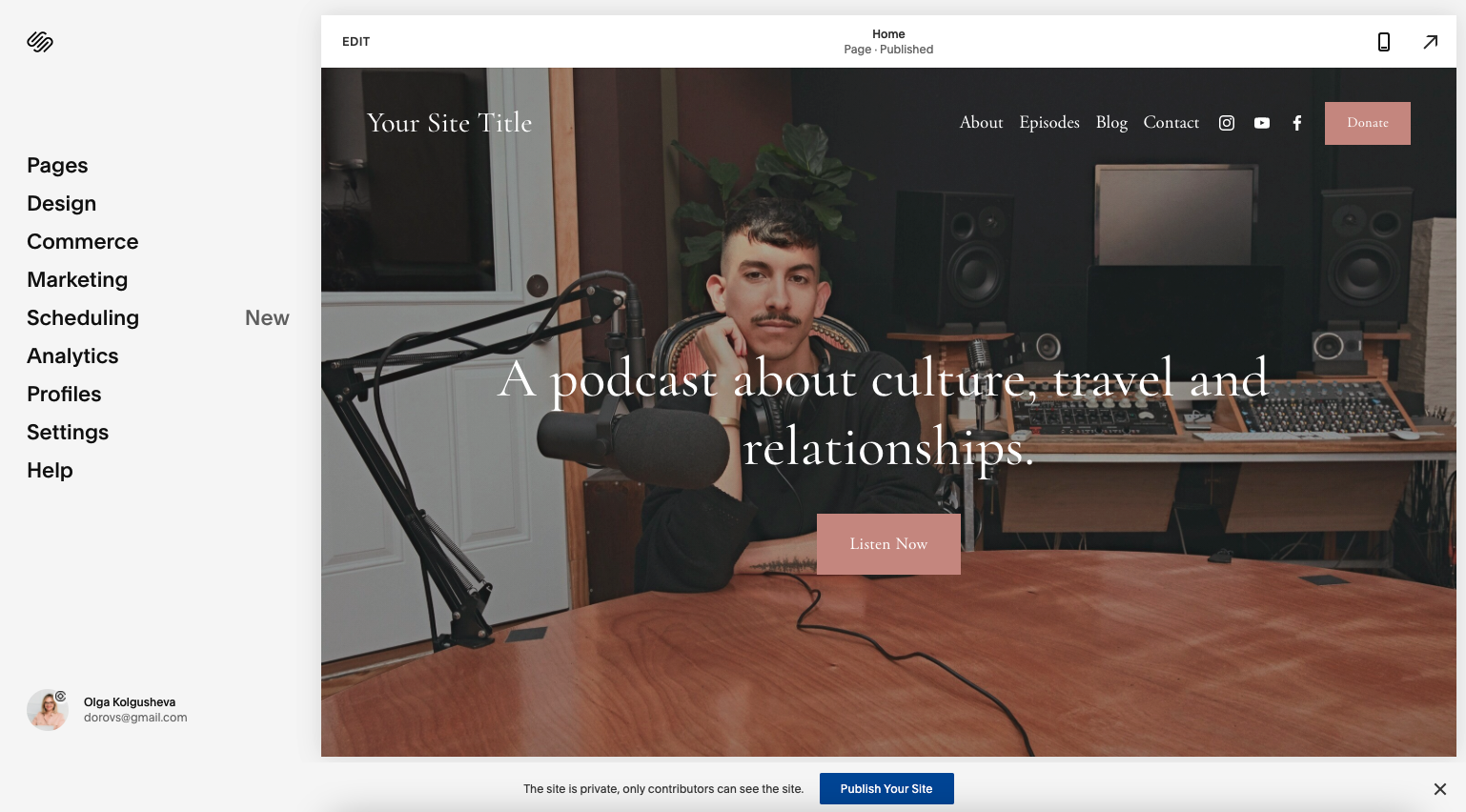This image is a screenshot from an advertising campaign, showcasing the accessibility features of a website design product. The focus of the ad is on creating accessible and user-friendly websites. Uploaded by Olga, whose Gmail address is visible beneath the image, this screenshot highlights a sample podcast website dedicated to culture, travel, and relationships. 

The website features a banner with the text "A podcast about culture, travel, and relationships" and provides an option for users to listen now. At the bottom, there is a notice stating, "This site is private. Only contributors can see the site," next to a prominent blue button labeled "Publish Your Site."

At the top of the screen, there is a placeholder text "Your Site Title" in white font, suggesting that the user has yet to input a custom title for their site. Additionally, there is a small "Donate" button adjacent to the title box, allowing visitors to contribute funds to the website. Overall, this screenshot illustrates a clean, user-focused interface designed to facilitate easy and accessible website creation.